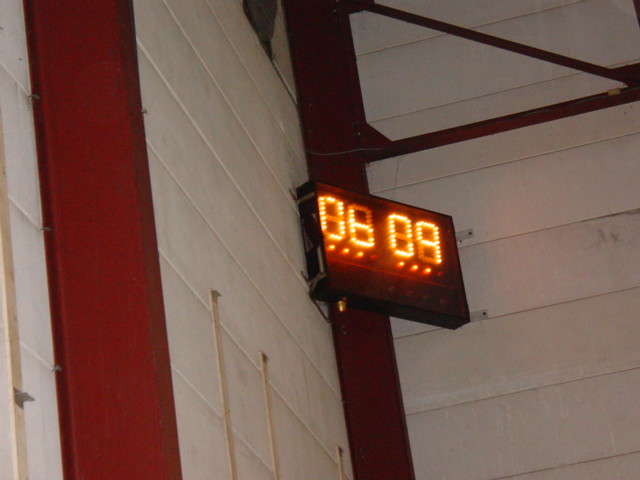The photograph depicts a low-light, indoor setting with a focus on the junction where two white, horizontal-paneled walls meet in a corner. Centrally positioned and slightly at an angle, there's a vertical rust-red I-beam, upon which a black rectangular digital scoreboard or time clock is mounted. The illuminated clock displays "0609" in bright red digits, accompanied by three small dots beneath the numbers. The left section of the image shows a prominent red column extending from the lower to the upper edge, while another horizontal beam projects from the central I-beam toward the right edge. Additionally, a diagonal structural piece connects to this horizontal beam near the right edge of the photo. Small screws and vertical tape-like features are visible along the support beams and walls, enhancing the industrial aesthetic of the scene, likely within a gymnasium or auditorium.